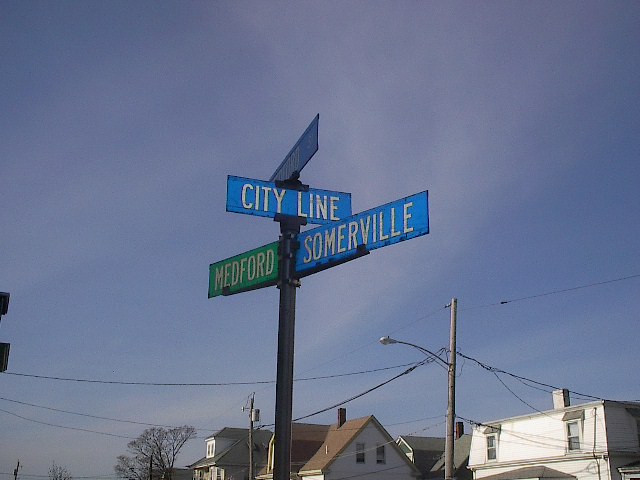In the image, a prominent street signpost stands tall, adorned with multiple street signs indicating various directions and locations. From the bottom, one sign reads “Medford” on one side and “Somerville” on the opposite side, both featuring white text on a blue background. Above this sign, another sign bears the label “City Line,” also in white text on a blue background. At the very top of the pole, there is an additional sign that is sharply angled, making its text difficult to decipher. 

The bottom left sign is distinguished by its green color, also with white text. The signs collectively serve to demarcate boundaries and direct travelers in what appears to be an urban neighborhood. In the backdrop, large, white-painted houses with varied roof colors stand prominently. Additionally, electrical wires stretch across the scene, connected to a utility pole, reinforcing the cityscape setting. Above, the sky is predominantly blue with a few thin, wispy clouds scattered across it, adding a serene touch to the otherwise bustling environment.